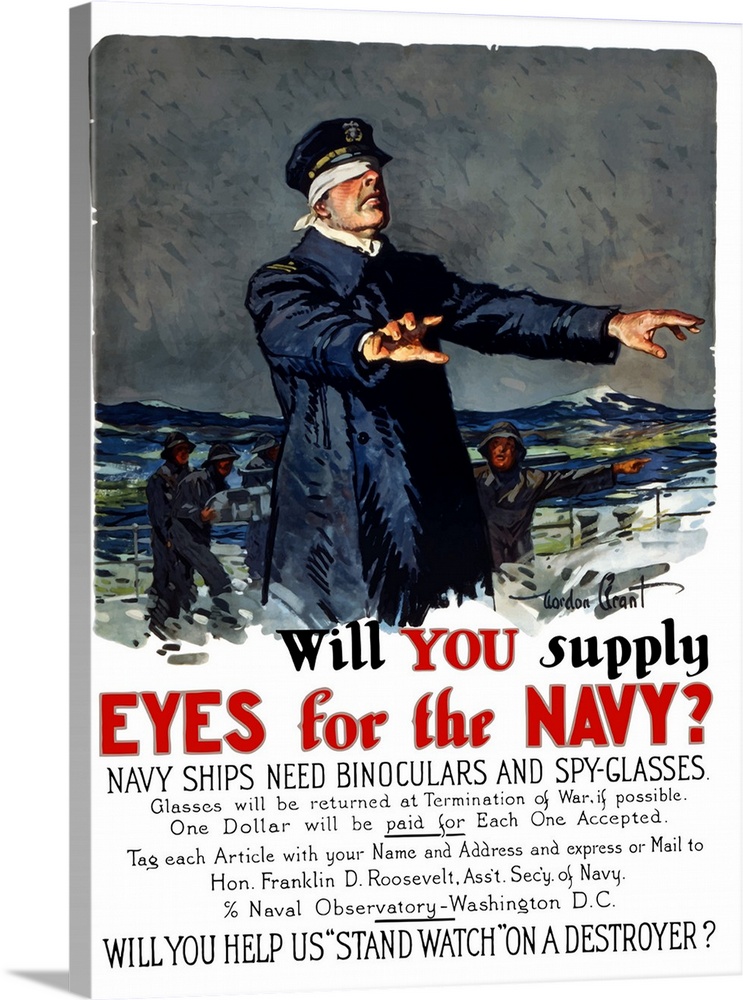The image depicts a historic poster from one of the World Wars. Dominating the foreground is a man dressed as a sea captain, adorned in a navy blue trench-style raincoat and a captain's hat with a gold emblem prominently displayed at the front. The captain's eyes are obscured by a white blindfold, and his arms are outstretched as if he is trying to feel his way forward. The backdrop of the poster features a tumultuous gray, stormy sky and a roiling blue sea dotted with whitecaps. In the background, several sailors are visible, standing against the railing of a ship.

The text on the poster, placed beneath the image, reads: "Will you supply eyes for the Navy?" The words "you" and "eyes for the Navy" are highlighted in red font. Following this, the text continues: "Navy ships need binoculars and spy glasses. Glasses will be returned at the termination of war if possible. One dollar will be paid for each one accepted. Tag each article with your name and address and express or mail to Honorable Franklin D. Roosevelt, Assistant Secretary of Navy, Care of Naval Observatory, Washington, D.C. Will you help us stand watch on a destroyer?"